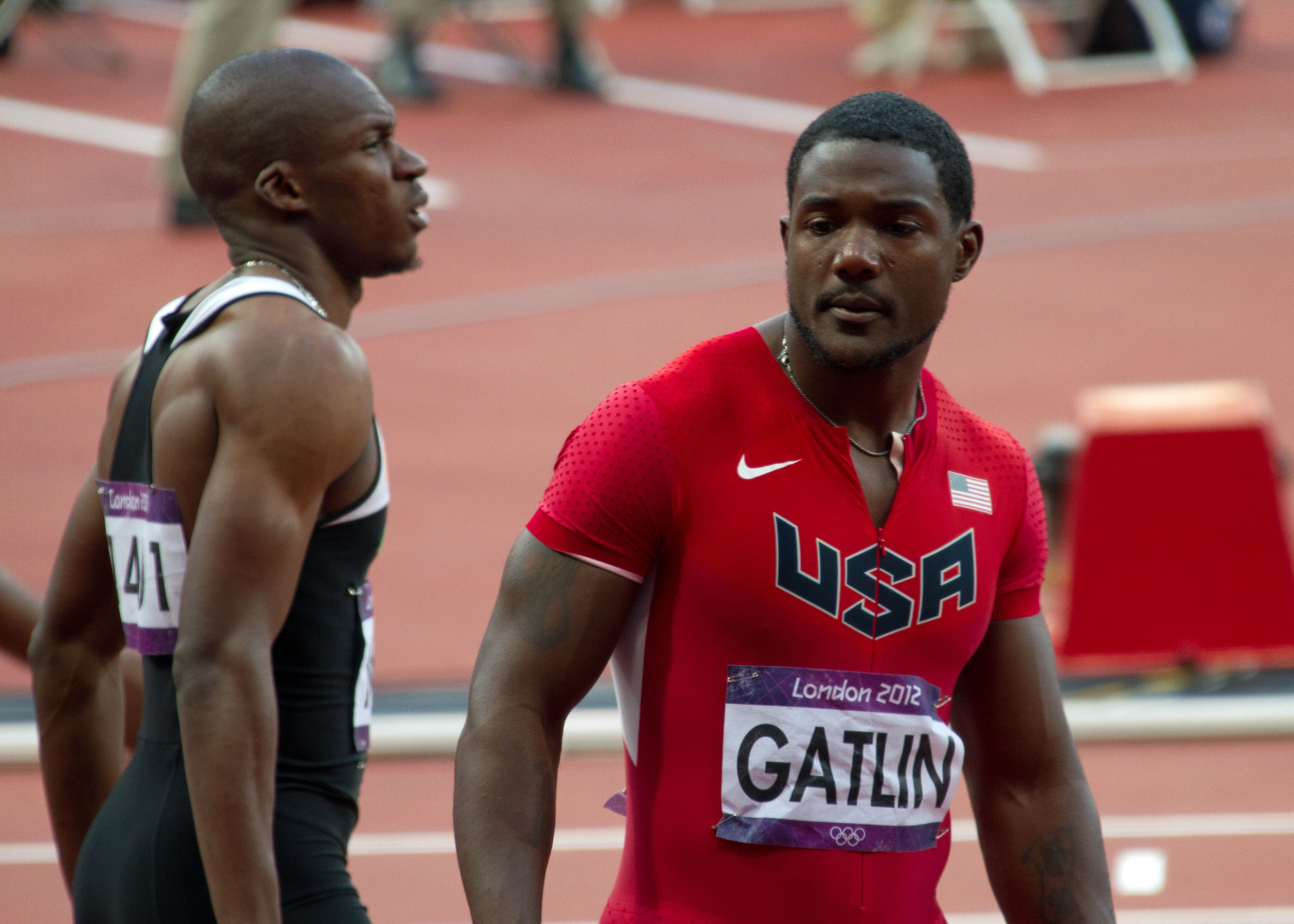The image captures two African-American men on a running track, seemingly Olympic sprinters. The man in the foreground is wearing a red Nike athletic jersey with short sleeves. The jersey features the American flag on his left shoulder and the Nike swoosh on his upper right shoulder. Prominently displayed across the chest is "USA," beneath which is a name tag on a white background that reads "Gatlin." Above the name tag, in purple text, it says "London 2012," and below it are the Olympic rings, indicating the setting as the 2012 London Olympics. He is glancing to his right at another athlete, who is clad in a black and white uniform. This second athlete has the number 41 on his back and also bears an Olympic tag. Both athletes seem to be either about to start or have just completed a race, with the running track visible in the background.